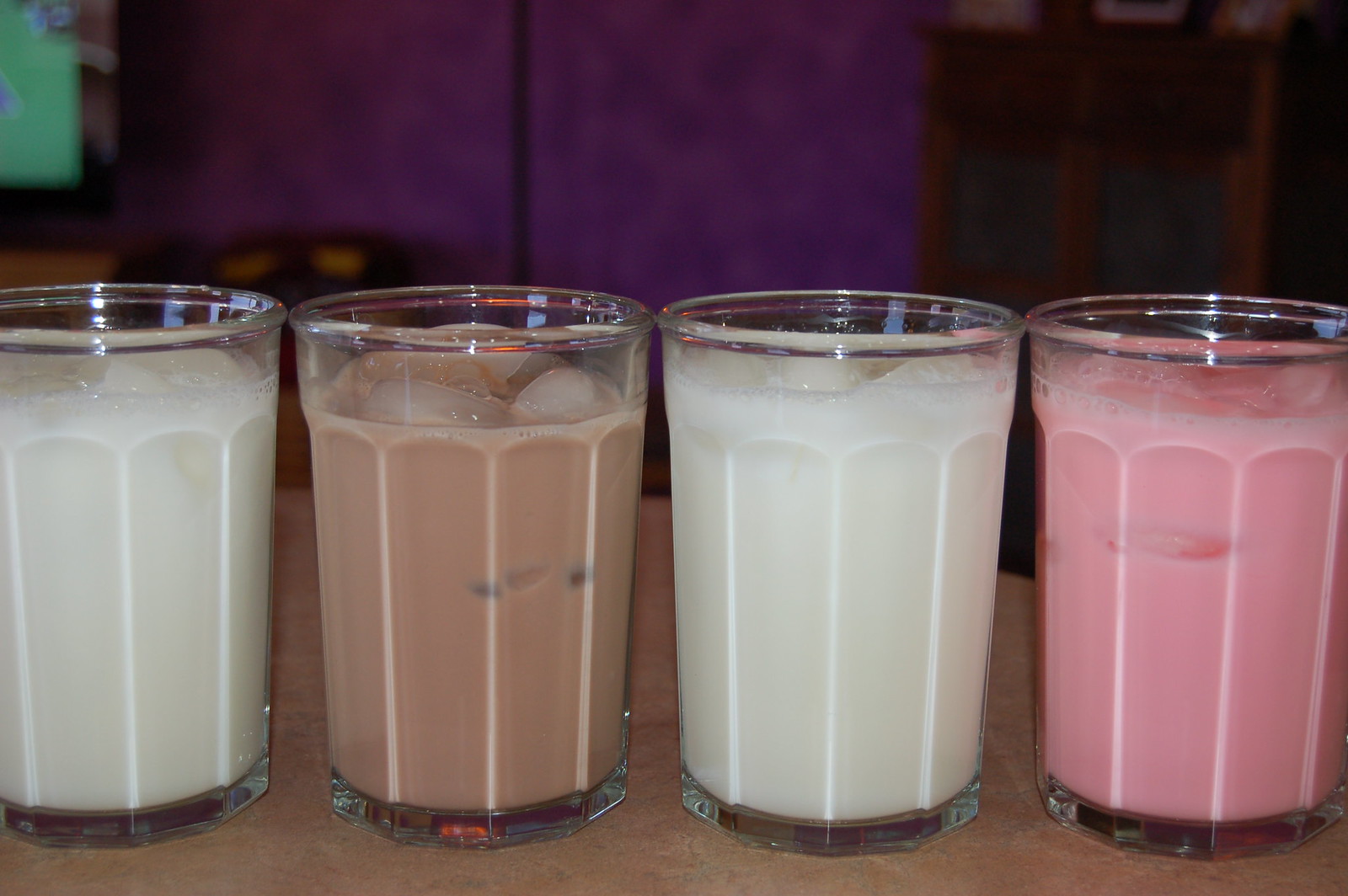This image features four short, clear glass cups arranged side-by-side on a brown wooden table, each filled with different kinds of milk drinks. From left to right, the first and third glasses contain white milk with ice cubes floating in it. The second glass is filled with chocolate milk, also with ice cubes, while the fourth glass holds pink strawberry milk topped with ice. The background reveals a purple wall with a visible dark brown area to the right and a small portion of a picture frame with a green hue on the left. The glasses are positioned closely together, and the image is zoomed in, capturing mainly the glasses and the tabletop.